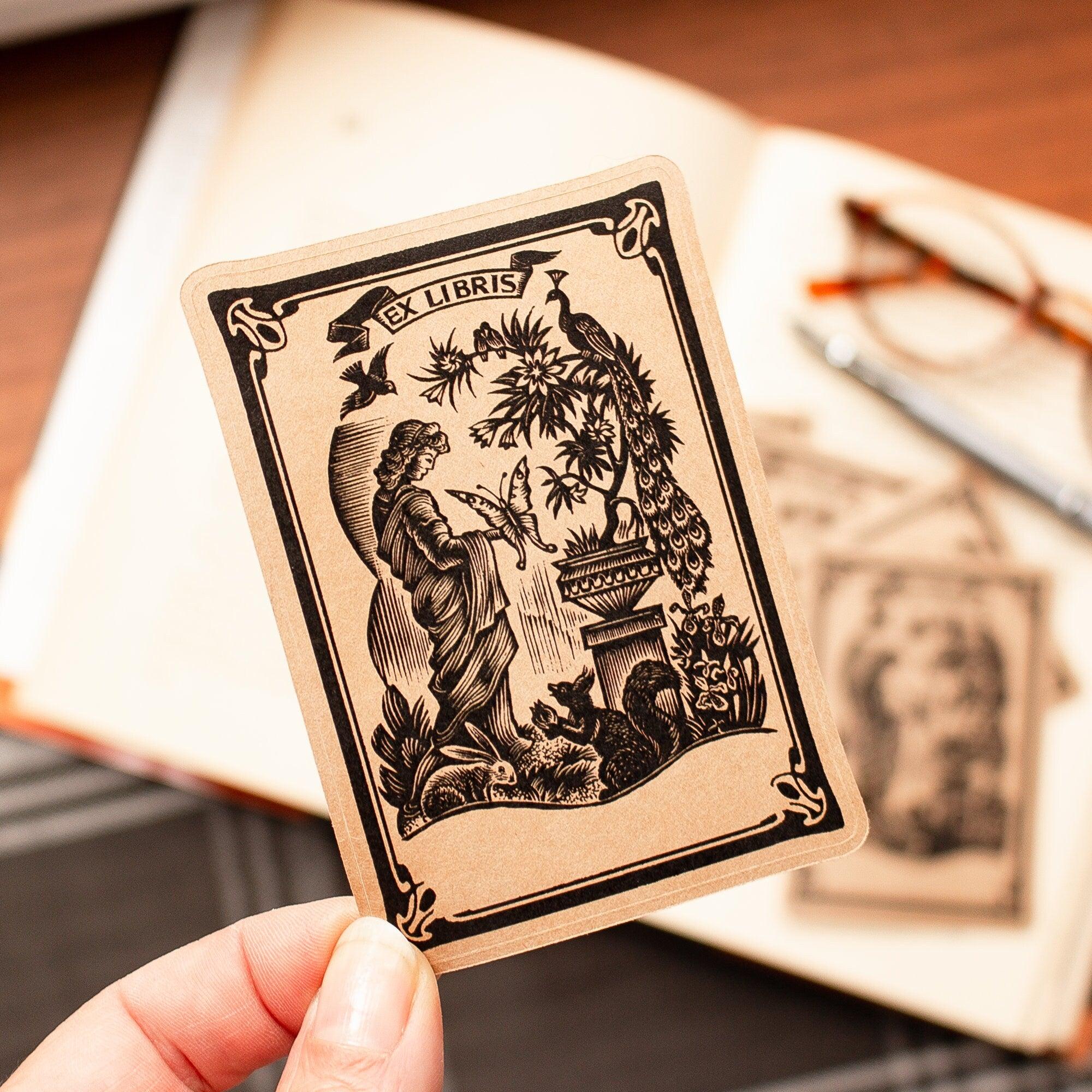This photograph is a highly detailed close-up of a person's two fingers holding a card, similar in size to a trading or tarot card, against a blurry background. The card itself is tan with a black border and a black banner displaying the text "Ex Libris." The illustration on the card features a woman with long hair, dressed in robes, holding a large butterfly. Surrounding her are intricate details including bunnies and squirrels at the bottom, and a tall garden plant with a peacock perched on it. In the background, out of focus, are additional cards, an open book resting on a brown wooden table, a pair of glasses, and a pen, all adding to the scene's rich and textured composition. The image emphasizes the clear, textured detail of the fingers, showing skin wrinkles and nail coloring, juxtaposed with the blurred elements in the background for a striking depth of field.